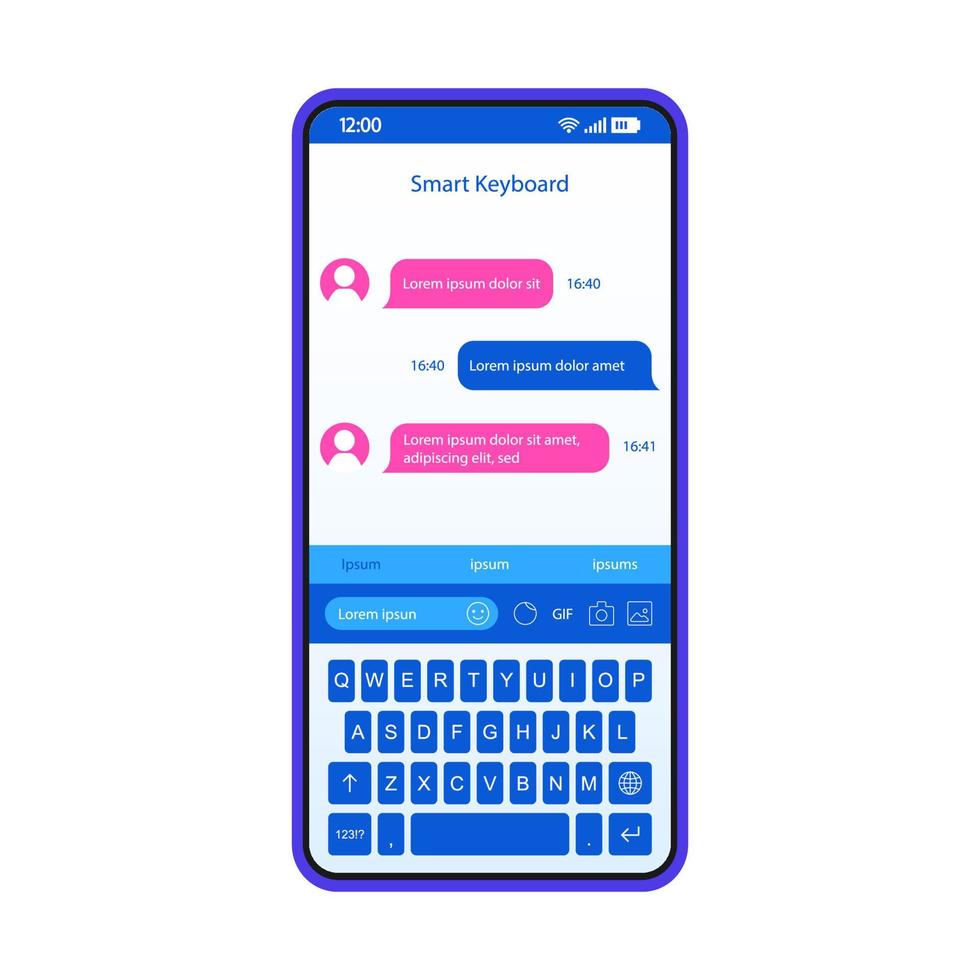The image features a detailed, stylized diagram of a smartphone with a white background. The phone itself has a purple trim and prominently displays its screen. At the top of the screen, the interface indicates the current time as 12:00, along with status icons for WiFi, volume, and battery life, which is notably at 2%. The main portion of the screen highlights a blue smart keyboard interface at the bottom with white letters. Above the keyboard, there's a conversation thread with placeholder "Lorem Ipsum" text. The first message, encased in a pink circle with a white silhouette of a person, reads "Lorem ipsum dolor sit" and is timestamped at 16:40. This is followed by a blue message bubble with white text that says "Lorem ipsum dolor omit," with a final pink message bubble stating "Lorem ipsum dolor sit omit, aperesciem elit sed." The bottom section also features functions for autocorrect, text input, smiley face, stickers, GIFs, taking a photo, sending a photo, and typical keyboard options including shift, enter, and numbers.